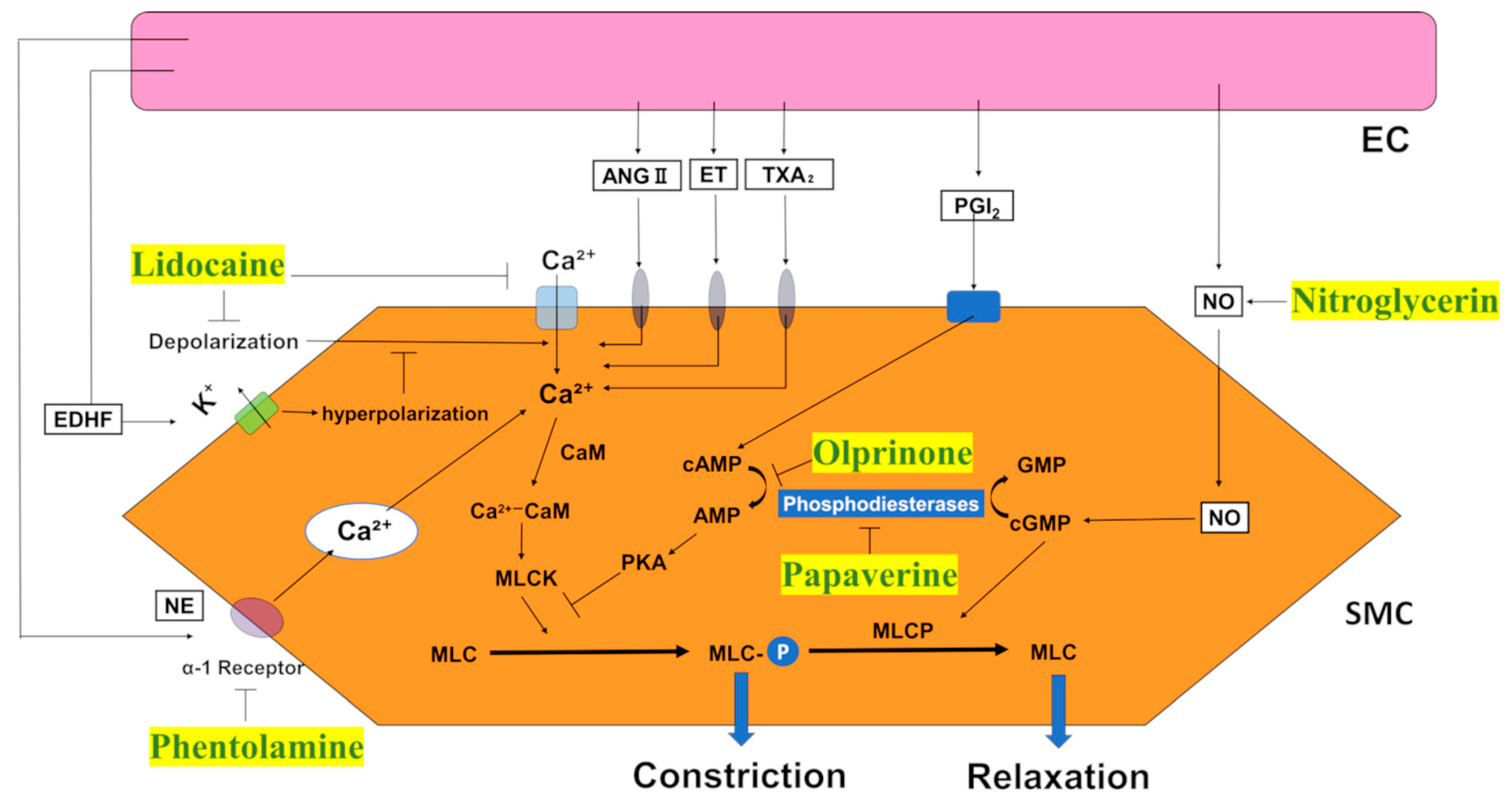The image is a scientific diagram illustrating a complex biochemical process involving Lidocaine, Nitroglycerin, and Phentolamine, among other chemical compounds. The diagram is set against a white background with a thin pink rectangle at the top and a prominent orange hexagon at the bottom. Within the hexagon, various chemical compounds and elements are interconnected by arrows, indicating a flow of reactions or interactions. Key terms such as depolarization, hyperpolarization, constriction, and relaxation are included, implying a focus on physiological processes. Lidocaine, known for its pain-relieving properties, is located at the top left of the diagram, while Nitroglycerin, a vasodilator, is positioned at the top right. Phentolamine is found at the bottom left, contributing to the complex web of interactions depicted. The diagram uses a variety of colors—orange, blue, and yellow—to differentiate various elements and processes, all hinting at a probable application in cardiac or vascular physiology.